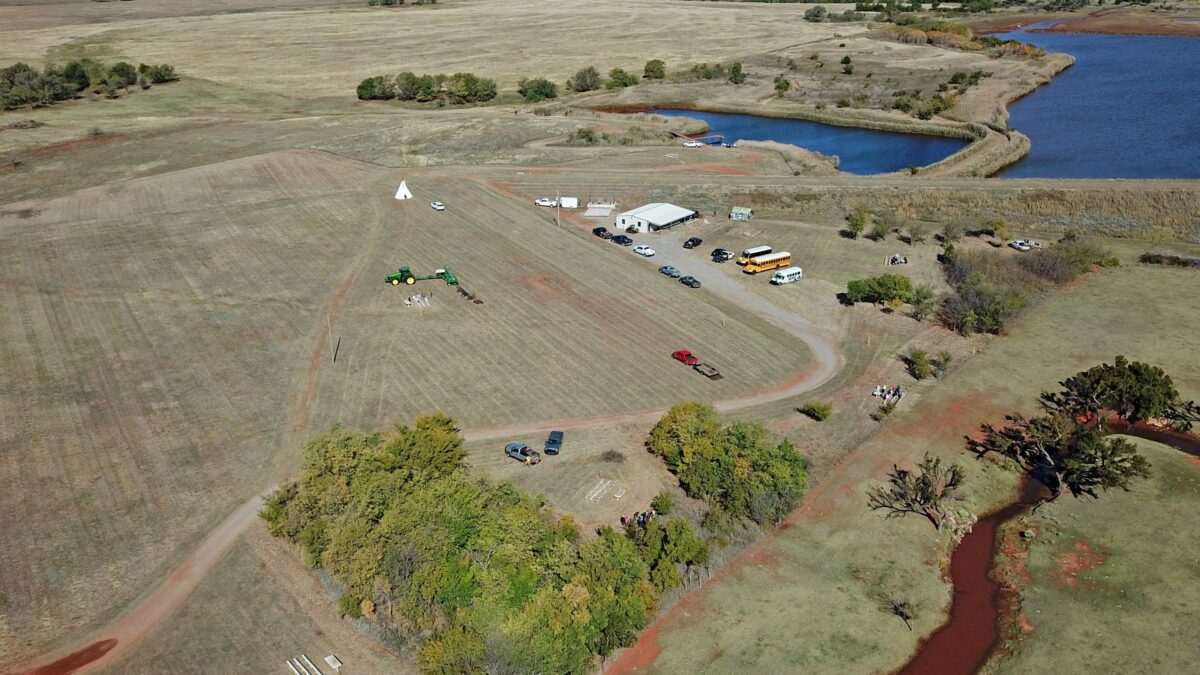This detailed aerial photograph captures an expansive farmland landscape with distinct features visible across the image. The primary focus is a patchwork of farming fields in varying shades of light gray and light green, meticulously arranged in rows. The fields stretch out across the land, interspersed with multiple clumps of trees - some positioned to the left, others in the middle, and groves of light green trees towards the front.

Prominently, there is a concentration of vehicles near a white building, potentially a hangar or parking area, situated on the middle-right side. Around this building, there are approximately 15 vehicles, including an orange or yellow bus, a white bus, and a notable green tractor with white wheels, as well as a red truck pulling a trailer.

To the top right, there is a body of water with dark blue hues, resembling a lake. On the bottom right, a brown stream curves gently from the middle right towards the bottom center, flanked by trees. Interestingly, there is a white teepee noticed within the field. 

The farmlands are clearly visible due to the aerial perspective, making it evident that this is a real photograph despite initial ambiguities about its authenticity. This panoramic view provides a comprehensive look at a rural area dedicated to agriculture, with various vehicles and structures adding to its dynamic scenery.